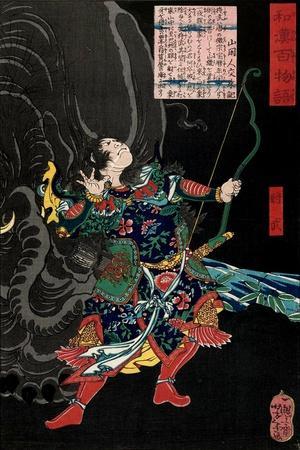The image is an intricately detailed Asian-style painting set against a black background, depicting a warrior in elaborate Japanese attire. The warrior, garbed in a navy blue robe adorned with floral patterns, gold, and green embroidery, wears striking red boots and tights. He is equipped with a green bow and a matching green sword tucked at his side, alongside a protective shield on his arm. His belt is adorned with various small items, emphasizing his detailed and practical ensemble. The warrior gazes upward with a tense expression, and his open hand suggests a sense of impending doom. Enveloping or emanating from him is a mystical, smoky octopus-like creature, adding a surreal and ominous atmosphere. At the top of the image, a white box with Asian script, likely Chinese, is prominently displayed, while the right corner features another red rectangular box with Asian characters. In the bottom right corner, there is a peanut-shaped image containing more Asian writing.